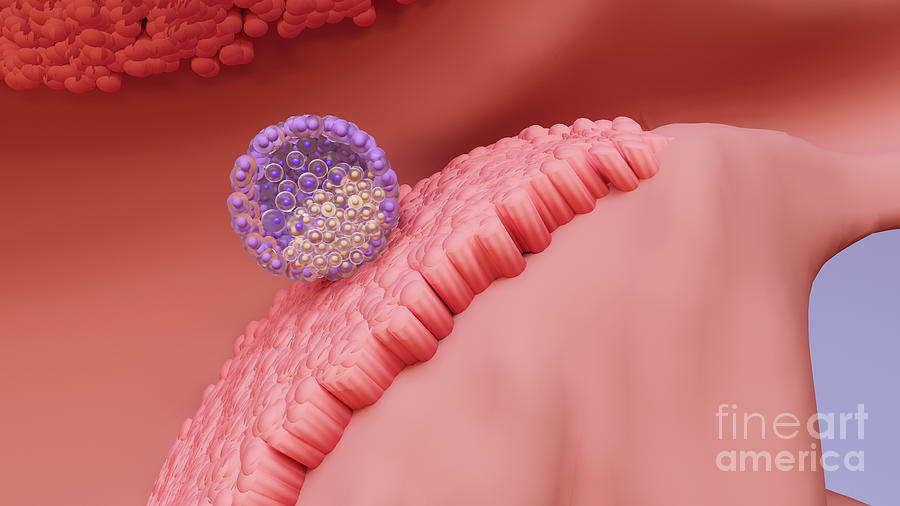This intricate image appears to be a virtual or 3D animated representation, possibly of some cellular or tissue structure. The backdrop is a reddish-brown hue, evoking inner body environments. At the top left, there's a cluster of small red circular objects, resembling cells. Dominating the right-hand side is a large pink expanse, which is partly smooth and partly textured with bumpy, flesh-like structures. A notable feature is a purple circular object adorned with an array of smaller purple and white orbs, creating a striking concentric pattern. Inside this circle, there are additional tiny circles in gold, blue, and purple, suggesting some complex biological formation. The scene is accented with a few orange spheres at the very top. On the bottom right corner, a watermark reads "Fine Art America" in light white font, resting between the fleshy part and a grayish area.